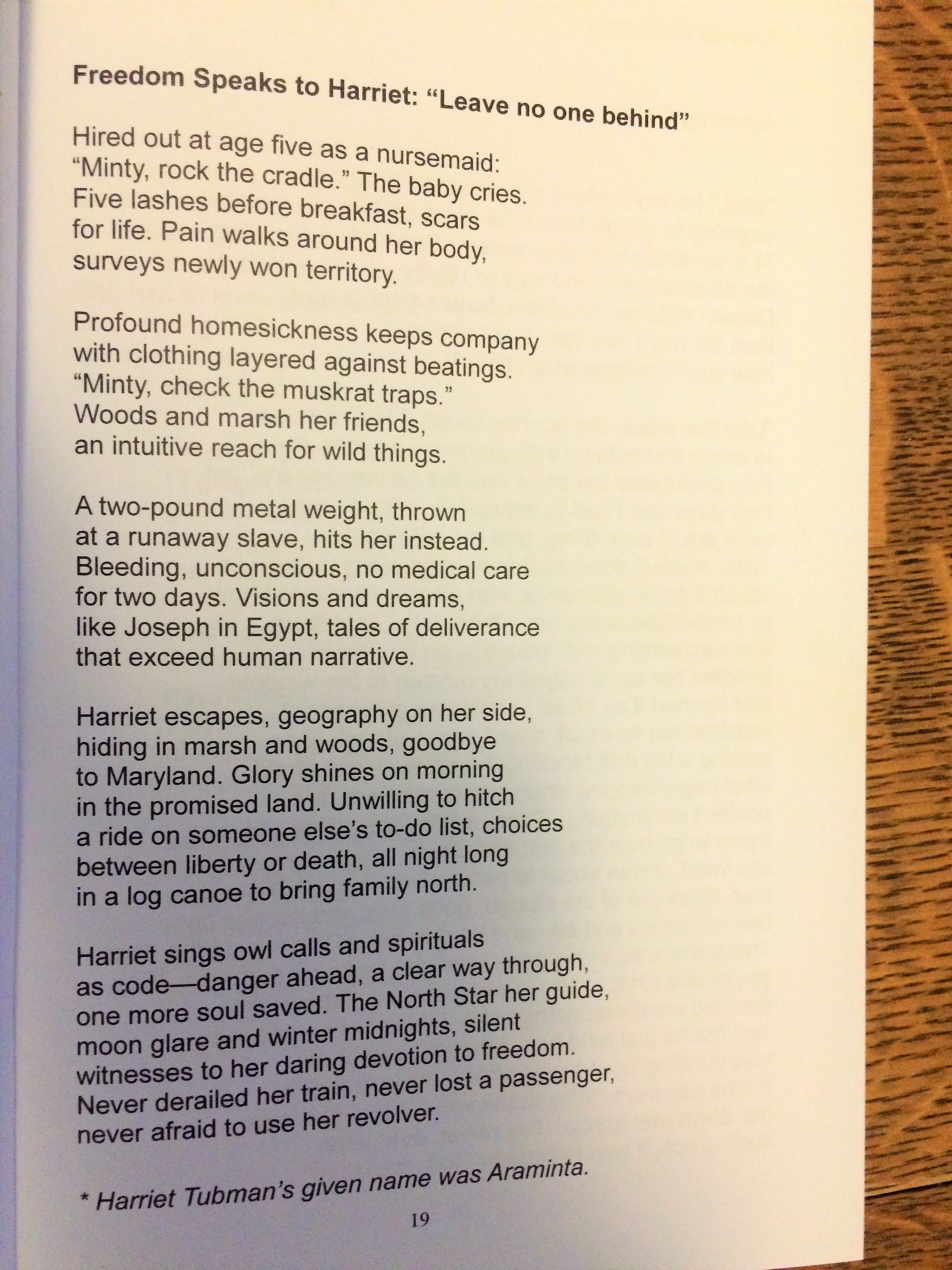The image is a color photograph of an open book page, displaying a poignant poem titled "Freedom Speaks to Harriet, Leave No One Behind," dedicated to Harriet Tubman. The page, numbered 19, features black text on a white background and the book rests on a dark brown wooden table. The bold title at the top is followed by stanzas recounting Harriet Tubman's harrowing experiences: being hired out as a nursemaid at age five, enduring severe punishment and permanent scars, dealing with profound homesickness, and befriending the woods and marshland. A significant event describes a two-pound metal weight hitting her instead of a runaway slave, leaving her bleeding and unconscious without medical care for two days. The narrative captures her visions and dreams akin to Joseph in Egypt, symbolizing tales of deliverance beyond human understanding. An asterisk at the bottom notes Harriet Tubman's given name was Araminta.